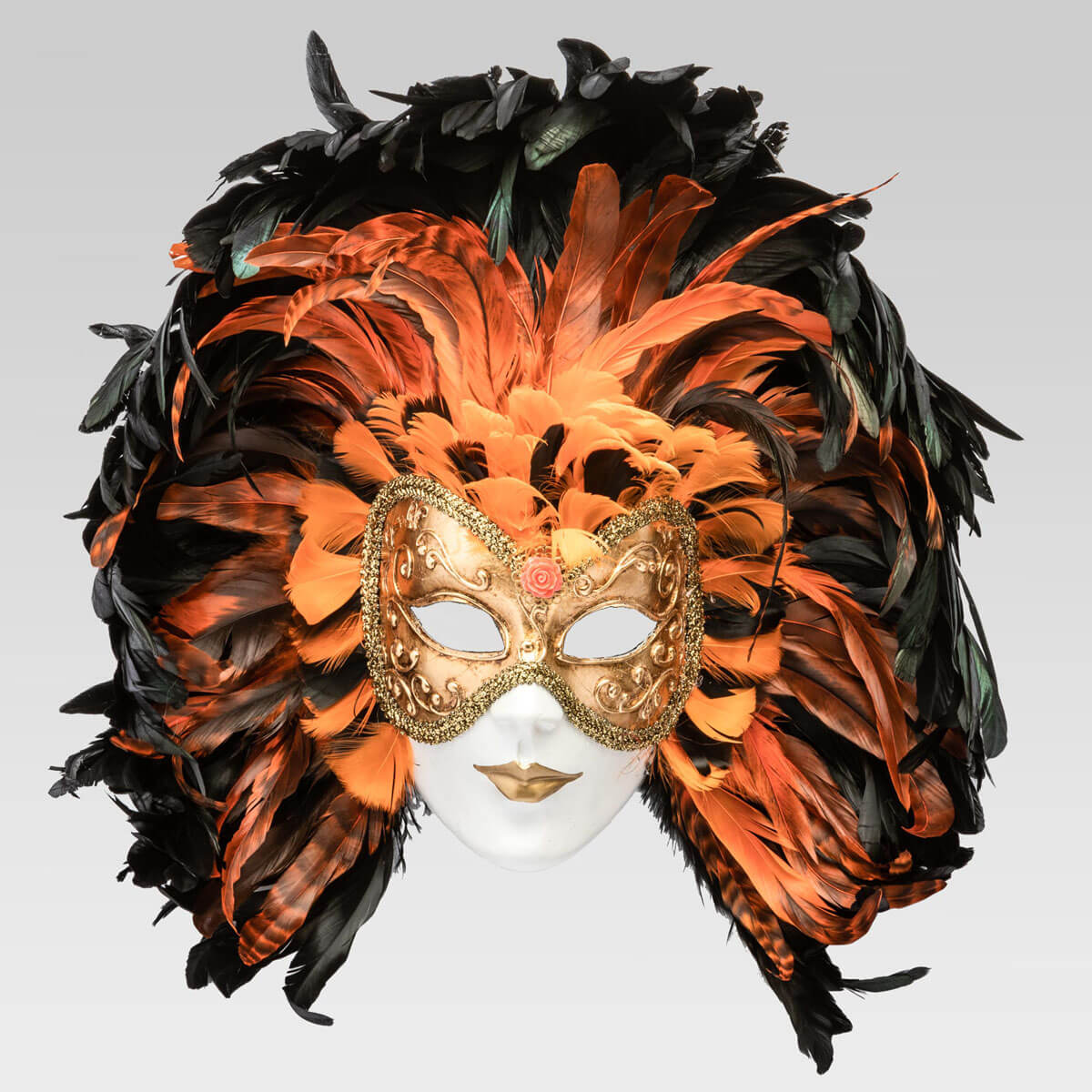The image depicts an elaborate artist's sketch, possibly of a mannequin, showcasing a highly ornate carnival mask. The mask, which appears to be made of gold or polished brass, is intricately designed in the shape of a butterfly with decorative scrolls and leaf motifs. It covers the face from just above the nose to the eyebrows and extends over the cheeks. The mask features eye openings and is accentuated with striking gold lipstick on the wearer. 

Surrounding the mask, a magnificent array of feathers spans outwards, ranging in color from vibrant orange to deep black. The feathers form large plumes that extend up over the head and around the sides, creating a halo-like effect that is about as wide as the skull. Some feathers even display orange and black stripes, adding to the rich texture of the composition. The background is light gray, which enhances the vividness of the mask and its feather adornments. Overall, the sketch presents a captivating and detailed portrayal of a festival mask in a lavish display of color and craftsmanship.